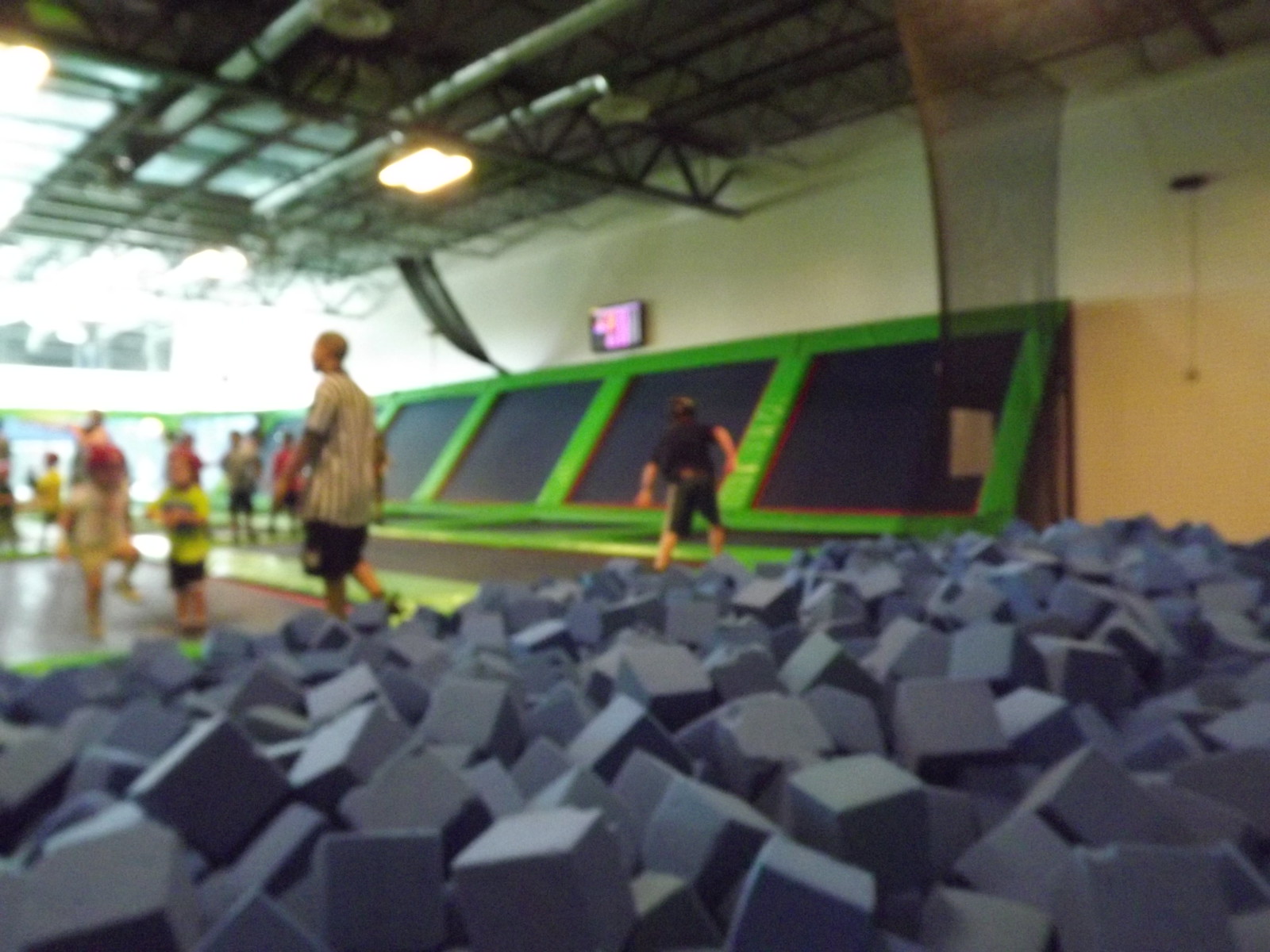This detailed image depicts a bustling indoor trampoline park designed for recreational activities such as jumping on trampolines and diving into foam pits. Dominating the left side and stretching towards the back are numerous trampolines, where two kids, one wearing a white shirt with yellow shorts and the other in a neon yellow shirt with black shorts, can be seen standing. To their right is a person dressed in a referee shirt and black shorts, likely an employee overseeing the activities.

A young man dressed in a black t-shirt and shorts is actively moving towards a series of diagonal trampolines set against a yellow wall, which are separated from the main wall by a green netting. This netting consists of square-shaped green padding and appears similar to trampoline material. The background shows additional blurred figures, creating a sense of a lively environment, though their activities are indistinct due to a bokeh effect.

The ceiling features a network of black metal beams, adding to the industrial yet organized appearance of the facility. In the foreground, there's a substantial pile of blue foam blocks, serving as a cushioned landing area for jumpers. The overall setting is vibrant and dynamic, filled with elements designed for physical engagement and fun.